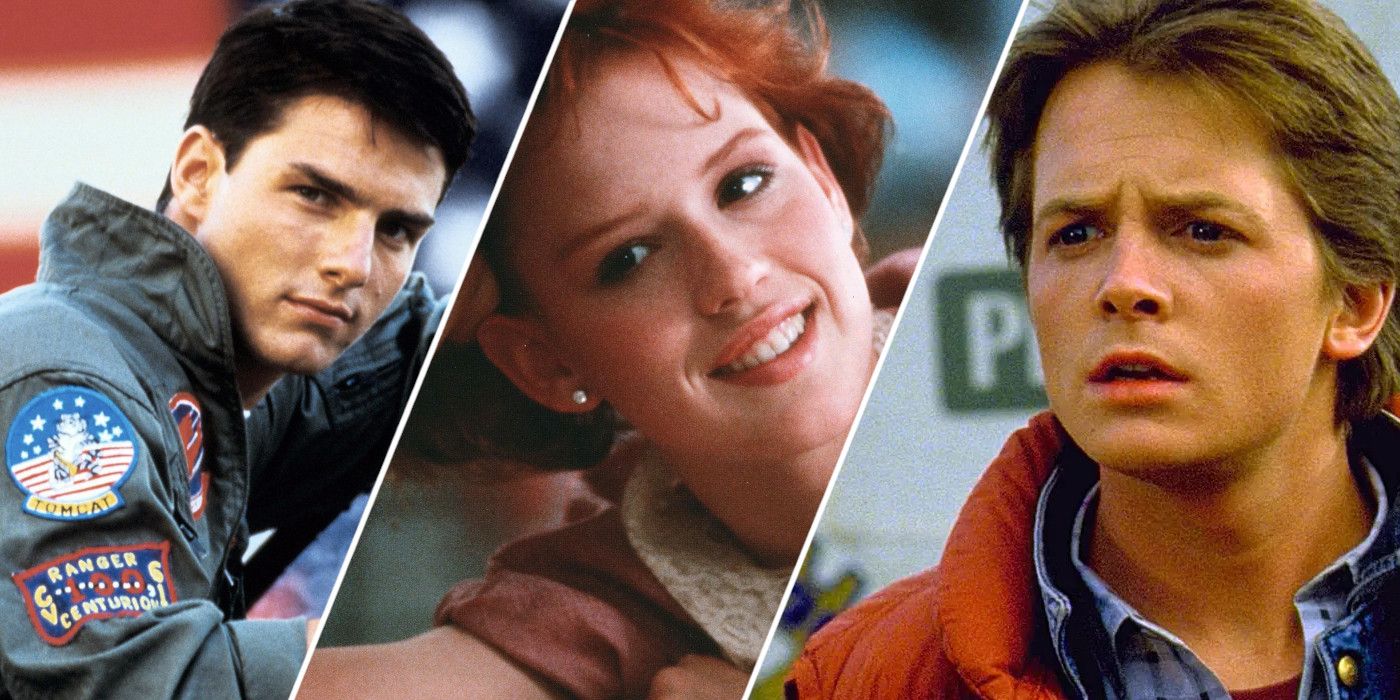This horizontal rectangular image, divided into three uneven sections by diagonal lines, features iconic 1980s celebrities each in a memorable role. On the far left, a young Tom Cruise is depicted in his "Top Gun" flight uniform, complete with patches that read "Ranger," "Centurion," and "Tomcat." His dark hair and youthful looks are unmistakable. In the center, an image of Molly Ringwald from "Pretty in Pink" captures her with auburn red hair, a smile, pierced ears, and wearing a pink or orangey outfit. On the far right, Michael J. Fox as Marty McFly from "Back to the Future" looks distressed, clad in his signature red vest over a denim jacket.